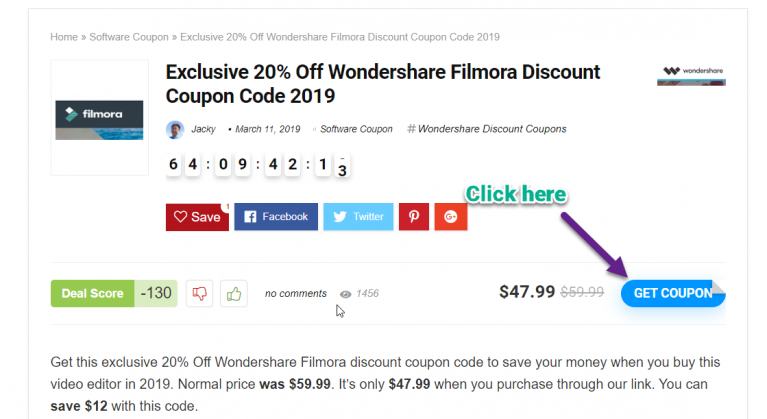The image is a screenshot of a web page advertising a discount on Wondershare Filmora software. At the top, the navigation bar includes categories labeled "Home," "Software," and "Coupon," followed by the headline, "Exclusive 20% Off Wondershare Filmora Discount Coupon Code 2019." 

Beneath this, prominently displayed in large black font on a white background, is a reiteration of the headline. To the left, the Filmora logo is clearly visible. Adjacent to the headline is a countdown clock indicating the time remaining for the offer, complemented by a set of options.

Following is a row of social media buttons for sharing the deal via Save, Facebook, Twitter, Pinterest, and Google+. Below these buttons is a prompt that says "Click Here," directing attention towards a blue "Get Coupon" button.

A green box underneath this section displays a "Deal Score" of -130, supplemented by thumbs-down and thumbs-up buttons for user feedback, with a note that there are "No Comments." To the right of this, the discounted price of $47.99 is shown.

Further down the page, an explanatory note highlights the savings: "Get this Exclusive 20% Off Wondershare Filmora Discount Coupon Code to save your money. When you buy this video editor in 2019, the normal price was $59.99. It's only $47.99 when you purchase through our link. You can save $12 with this code."